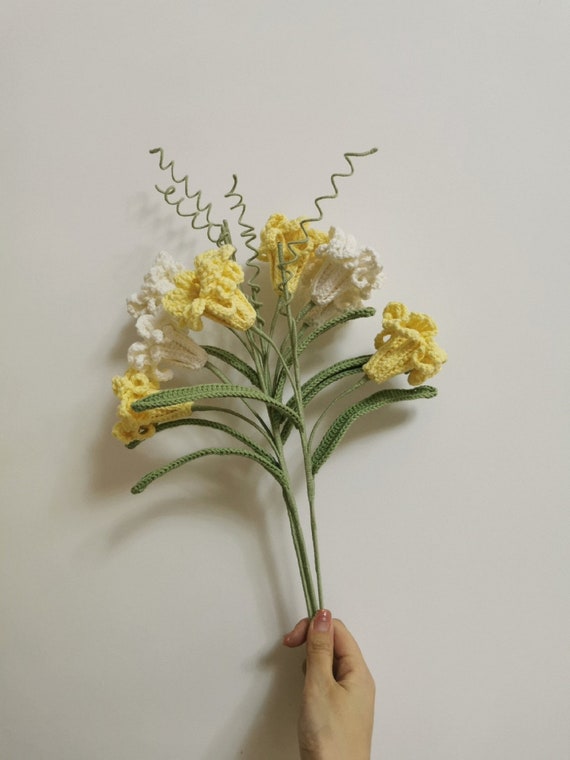The image showcases a professionally crafted bouquet of intricately knitted or crocheted flowers, held by a hand with painted nails, possibly belonging to a woman. The bouquet consists of three or four green stems adorned with a total of seven flowers—four yellow and three white. The stems are embellished with detailed leaves and vines, all in a greenish hue. The quality of the craftsmanship is exceptional, making the flowers appear almost real at a glance. The background features a plain white wall, accentuating the vibrant colors of the bouquet while highlighting the meticulous work put into each element of the art piece.